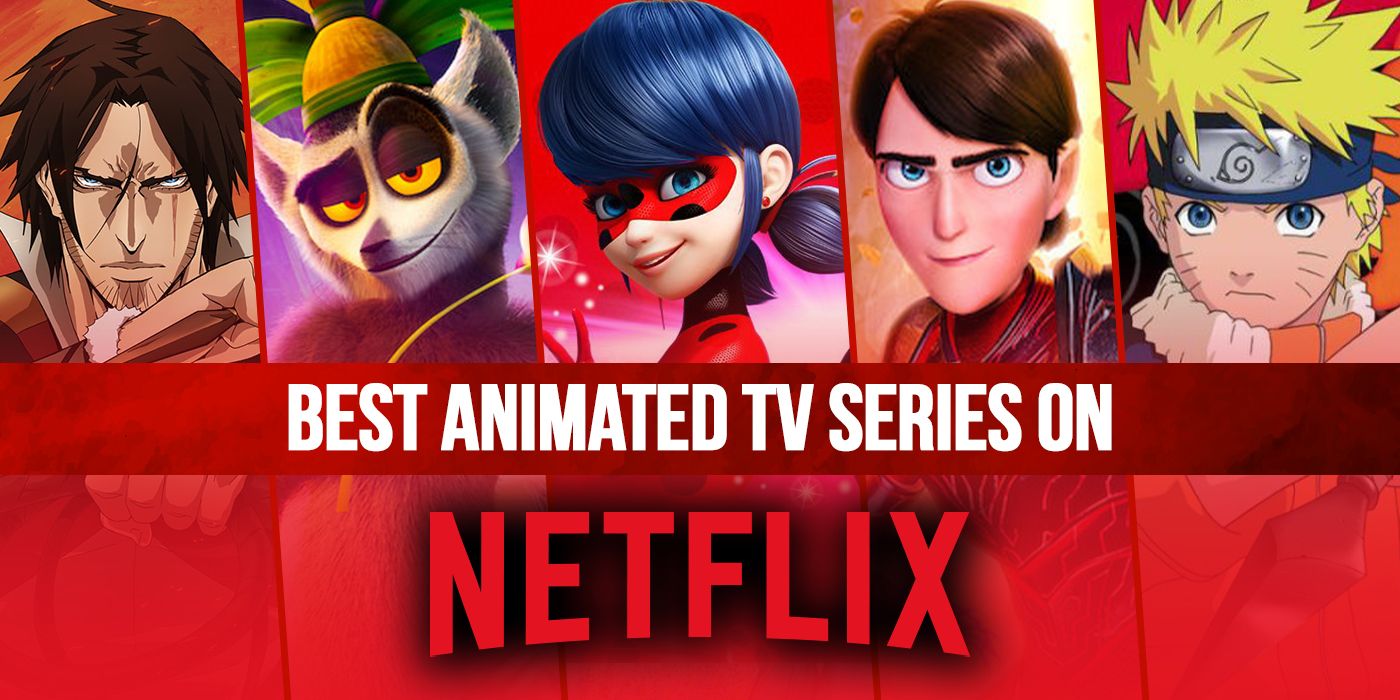The advertisement for Netflix prominently showcases the slogan "Best Animated TV Series on Netflix" in white text on a red ribbon, positioned just above the distinctive Netflix logo in permeating red text with a shadowy black border. Above this text, five distinct characters from various animated or 3D animated movies and shows are displayed. On the far left, the serious figure holding a whip is Trevor from Castlevania, a white male with longer brown hair. Next to him is a smirking lemur, followed by a masked woman in a colorful costume. The fourth character is another white male with brown hair and blue eyes, glancing knowingly at the viewer. Finally, on the far right, we see Naruto with his blonde hair and headband. The background features a red transparent field, highlighting the animated characters above and seamlessly integrating with the bold Netflix branding below. Each costume varies in color, from red and brown to cream and orange, enhancing the vibrant and dynamic visual appeal of the advertisement.